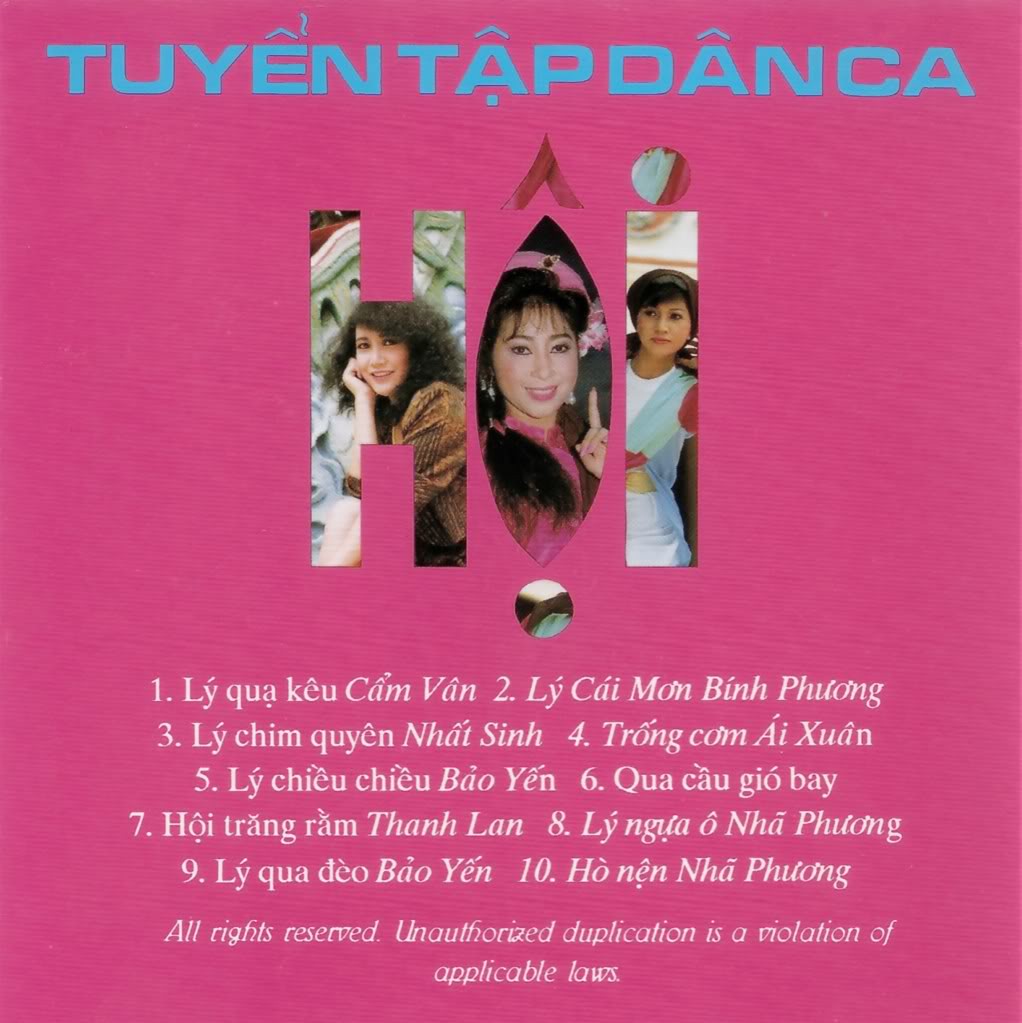The image appears to be a vibrant Instagram post with a hot pink background, resembling a vinyl album cover. At the top, blue text reads "Twintapdansa H-O-I," where each of the letters H, O, and I contains a picture of one of three young women of Eastern descent, seemingly in their twenties. Below this, in smaller white text, are ten names or song titles listed in what looks like the Tagalog language. At the bottom, there is an English disclaimer stating, "All rights reserved, unauthorized duplication is a violation of applicable laws."